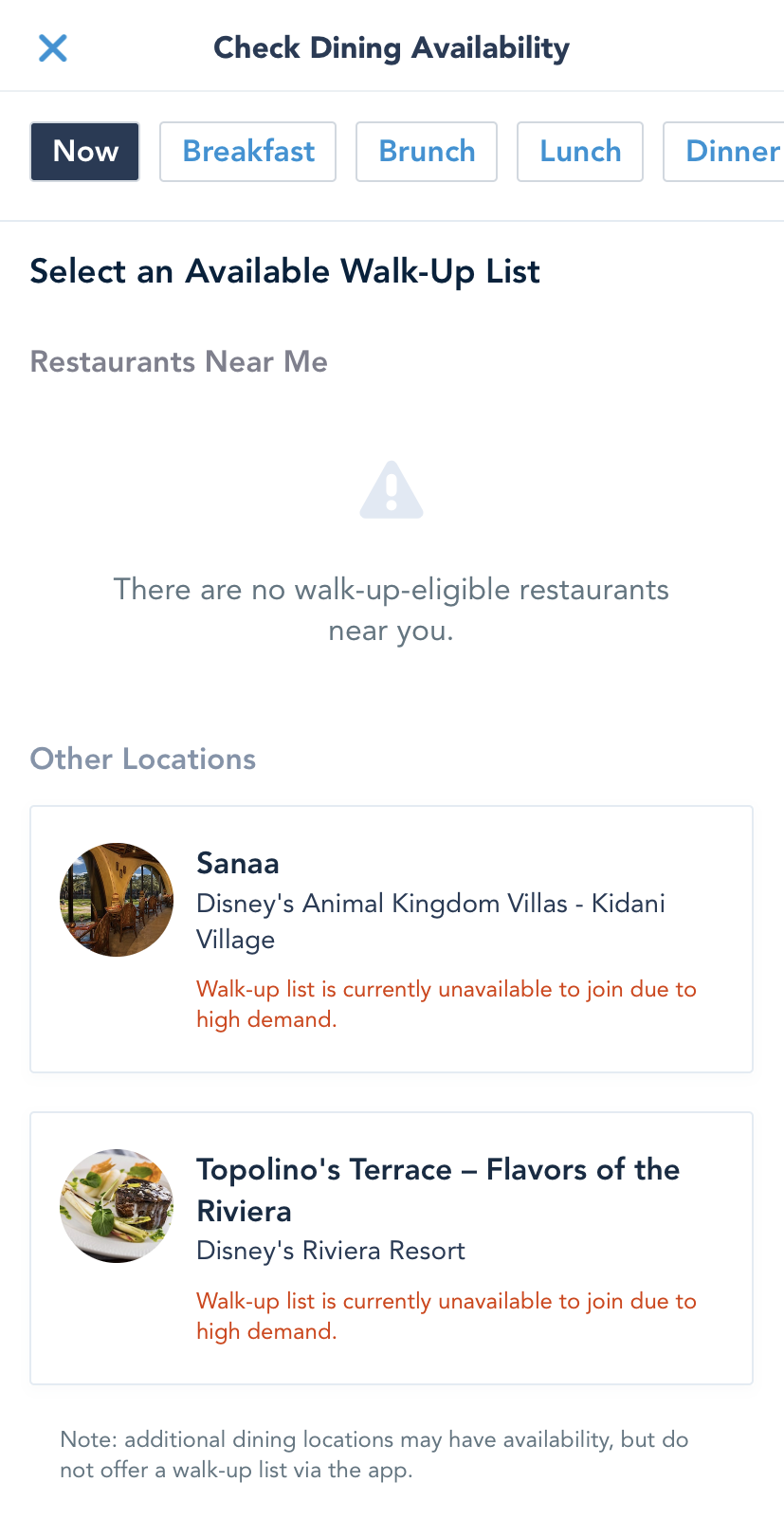This is a color image of a pop-up box likely from a website or app interface related to dining reservations. The background is predominantly white with mostly black text. In the upper left-hand corner, a blue "X" is visible for closing the pop-up. Next to it is text that reads "Check Dining Availability." Below this title, a thin black horizontal line separates it from the rest of the content.

The pop-up features several selectable options. On the left-hand side, a black box with white text indicates the currently selected option. The available meal options—Breakfast, Brunch, Lunch, and Dinner—are displayed in white with blue text, suggesting they are clickable links.

Beneath this, the text reads "Selected and Available Walk-Up List," followed by "Restaurants Near Me." An exclamation mark inside a gray triangle signals a notice: "There are no walk-up eligible restaurants near you."

Further down, two other dining locations are listed, each accompanied by small circular icons to the left, possibly depicting images of food or the respective restaurants. The first location is "Sanaa, Disney Animal Kingdom Villas - Kidani Village," with a note that the "Walk-Up List is currently unavailable to join due to high demand." The second location is "Topolino's Terrace – Flavors of the Riviera, Disney's Riviera Resort," which similarly indicates that the "Walk-Up List is also currently unavailable due to high demand."

At the bottom of the pop-up, there is a note stating, "Some traditional dining locations may have availability, but do not offer a walk-up list via the app."